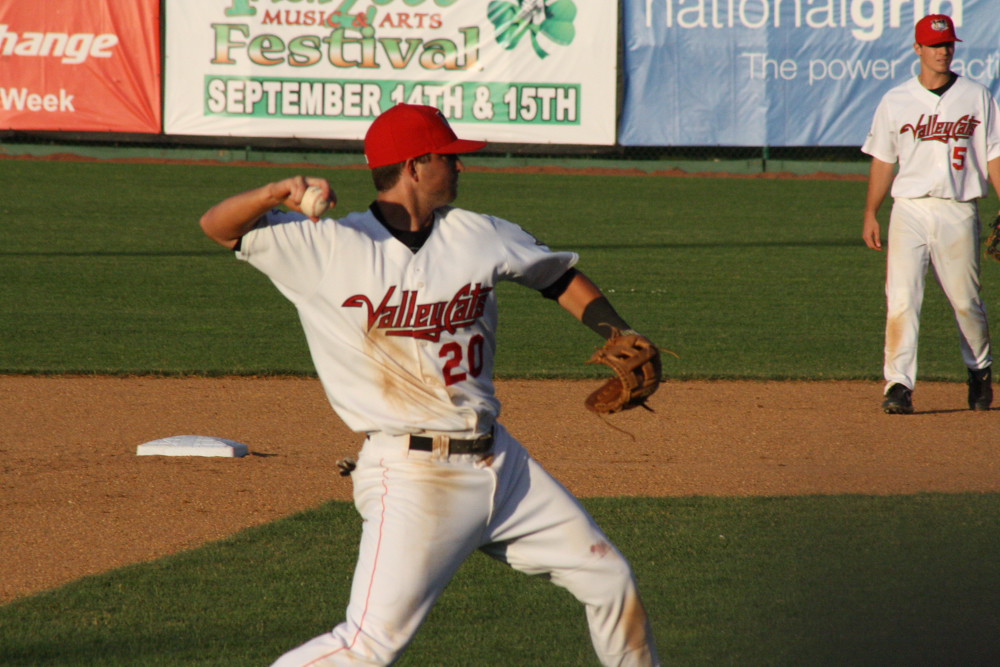This image captures a well-maintained baseball field where a minor league game is taking place, featuring the Valley Cats team. In the foreground, number 20, dressed in a white jersey with "Valley Cats" emblazoned in orange on the front and a red cap, is positioned to throw the ball across the diamond to the first baseman, number 5, who is also in a white uniform and red cap. The field is immaculate, with perfectly cut grass and pristine, brown dirt surrounding the base paths. The players' jerseys show signs of play, covered in dirt. In the background, a wall adorned with various banners and advertisements is visible. The banners include messages like "MUSIC AND ARTS FESTIVAL" scheduled for "September 14th and 15th" and a blue sign with the partially visible words "THE POWER." The scene is vibrant with details, from the sponges along the wall to the distinctive bright white bases, embodying the spirit and meticulous upkeep of minor league baseball.